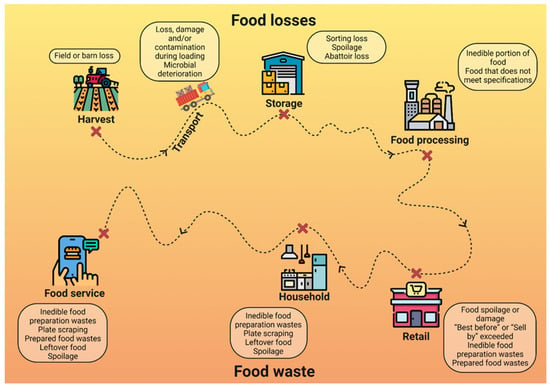This detailed diagram illustrates the journey and various stages where food losses occur, starting from harvest through to food service. At the top, "Food Losses" is prominently displayed in black letters, while the background color transitions from pale yellow at the top to light orange at the bottom.

The diagram maps out food loss through several stages, each represented by distinct icons. Beginning in the upper left corner, the diagram starts with harvest depicted by a farm icon, highlighting losses at the field or barn level. The journey continues to transport, marked by a truck icon, addressing issues like loss, damage, and contamination due to loading and microbial deterioration.

Following transport, the path moves to storage, represented by a blue warehouse icon, where sorting loss and spoilage can occur. Next is the food processing phase, signified by a factory icon, emphasizing inedible portions and food failing to meet specifications.

The road then curves down to the bottom right where retail is shown with a red store icon, underscoring food spoilage or damage and issues like exceeding best-before or sell-by dates. Moving leftward to the household stage, depicted by a kitchen icon, common issues include inedible food, preparation waste, and leftover spoilage.

Finally, at the bottom left corner, food service is represented by an icon of a person looking at a menu, indicating preparation waste, plate scraping, and leftover food spoilage. This comprehensive flow sheet effectively demonstrates the continuous cycle of food waste from harvest to the end consumer.